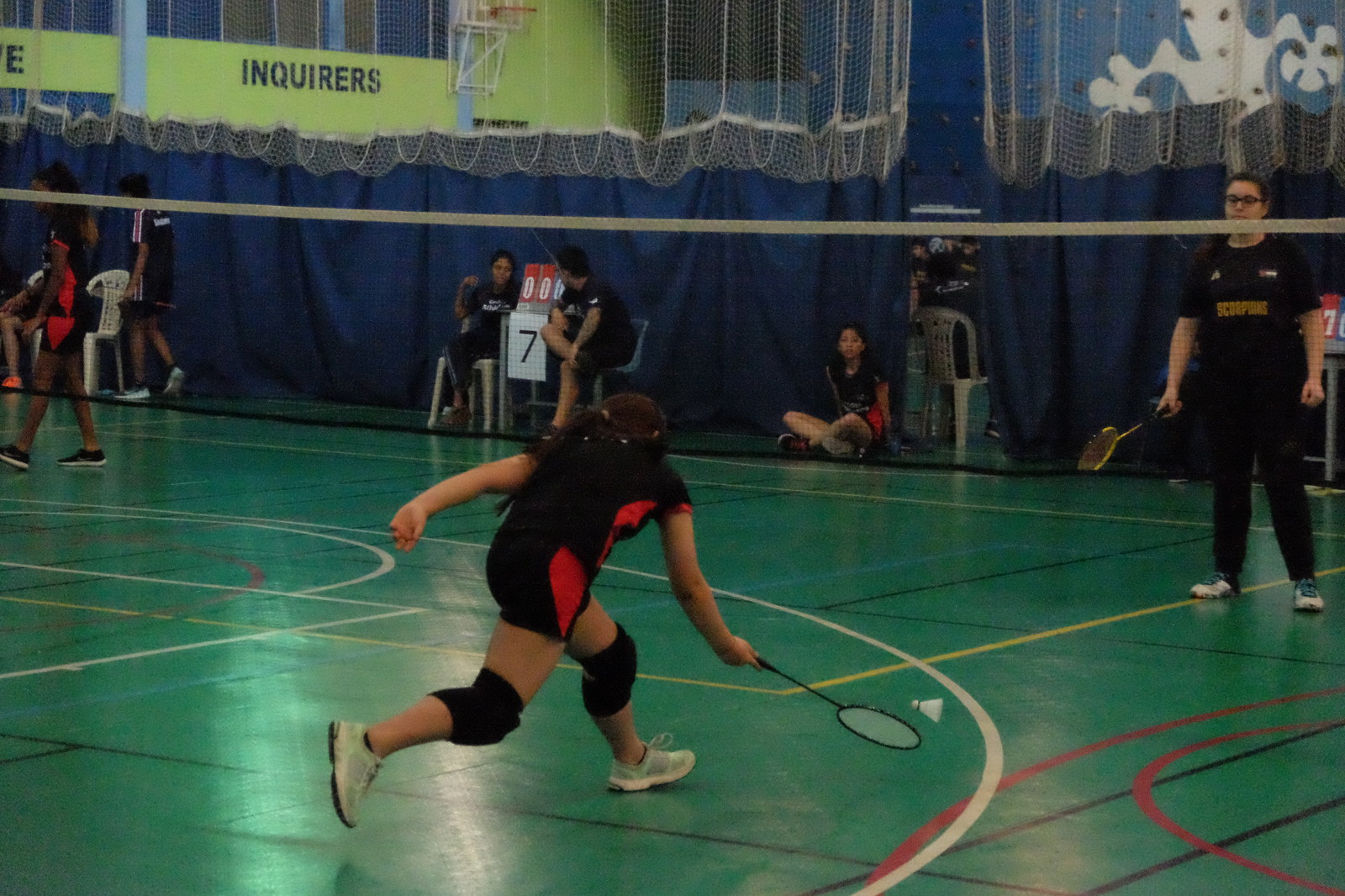The photograph captures an intense moment in a badminton tournament held inside a gymnasium with a bright green or teal floor marked with white, black, and red stripes. Central to the image is a woman in a blue and red uniform with knee pads and white sneakers, leaping forward with her left foot and stretching out her right hand, racket in hand, to strike a shuttlecock in mid-air. The opposing player, standing on the other side of the net and dressed in black clothing with gold lettering spelling "Scorpions," anticipates her move. Surrounding the court, several spectators sit and stand, attentively watching the match. In one corner, scorekeepers monitor the game, one displaying a number seven. The background features a dividing curtain splitting the gymnasium, adding to the scene's depth and focus on the sporting event.